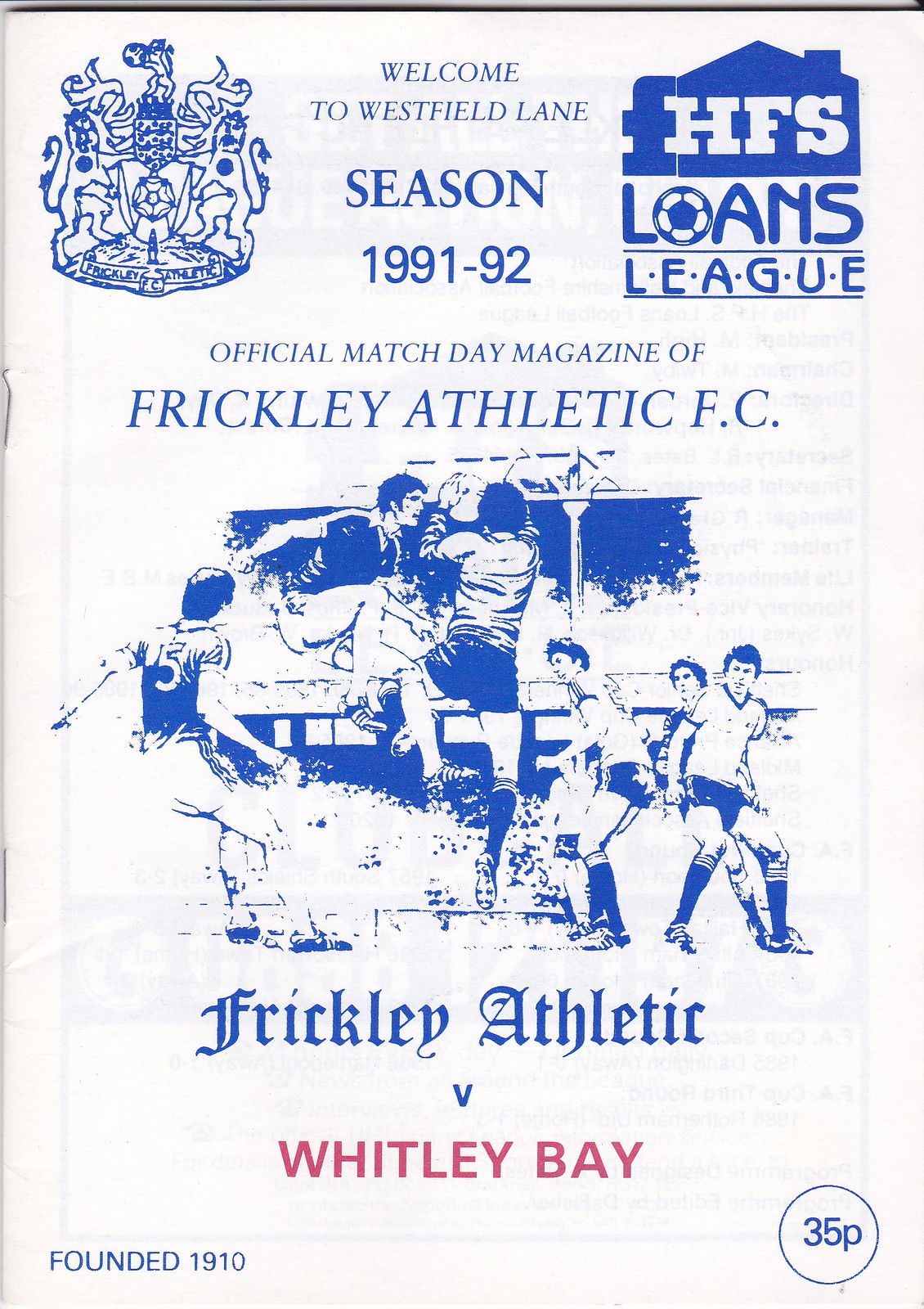The cover of this official match day magazine for the 1991-92 season of Frickley Athletic FC features a white background with predominantly blue print. It highlights "Welcome to Westfield Lane Season 1991-92" at the top. The upper left corner showcases the Frickley Athletic FC crest, while the upper right corner bears the HFS Loans League logo. Beneath these elements, there is a blue ink illustration depicting an intense moment in a football match where players are competing for the ball mid-air. The text below the image states "Frickley Athletic vs." with "Whitley Bay" in red. Additional details include "Founded 1910" in the bottom left corner and "35p" inside a blue circle in the bottom right corner.